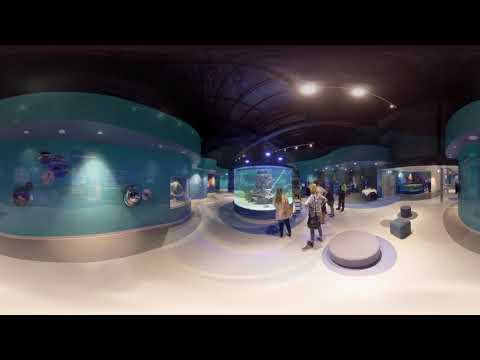The image depicts an aquarium or science museum with a slightly distorted perspective, making the normally straight lines appear curved. The scene features moderately crowded surroundings with several cylindrical displays that contain aquatic-themed exhibits. Slightly to the right of the image's center is a visible purple cushion, and beneath it, a darker circular cushion rests on the ground. Nearby, a dark green cube, which could also be a cushion, is present, along with a smaller, darker circle adjacent to it. 

In the foreground, two people are standing in front of a central aquarium tank that has a rocky structure inside. The person on the left wears a light brown jacket extending below the hips, dark pants, and has dark light brown hair shoulder-length. Next to them, another person wearing a light shirt with brown patterns, a black shoulder bag, and dark shoes stands, with blonde hair visible under two bright white ceiling lights. The ceiling itself is predominantly black, except for some areas appearing slightly purple and visible wiring.

The left third of the shot showcases a teal wall with a gray stripe at the top and an art piece consisting of black and purple colors at its center, illuminated by a light shining down. The floor beneath is white, contributing to the slightly dim overall illumination provided by the various small lights and the two main overhead lights. The gallery appears to extend into a hallway on the far right, suggesting further displays and exhibits for visitors.